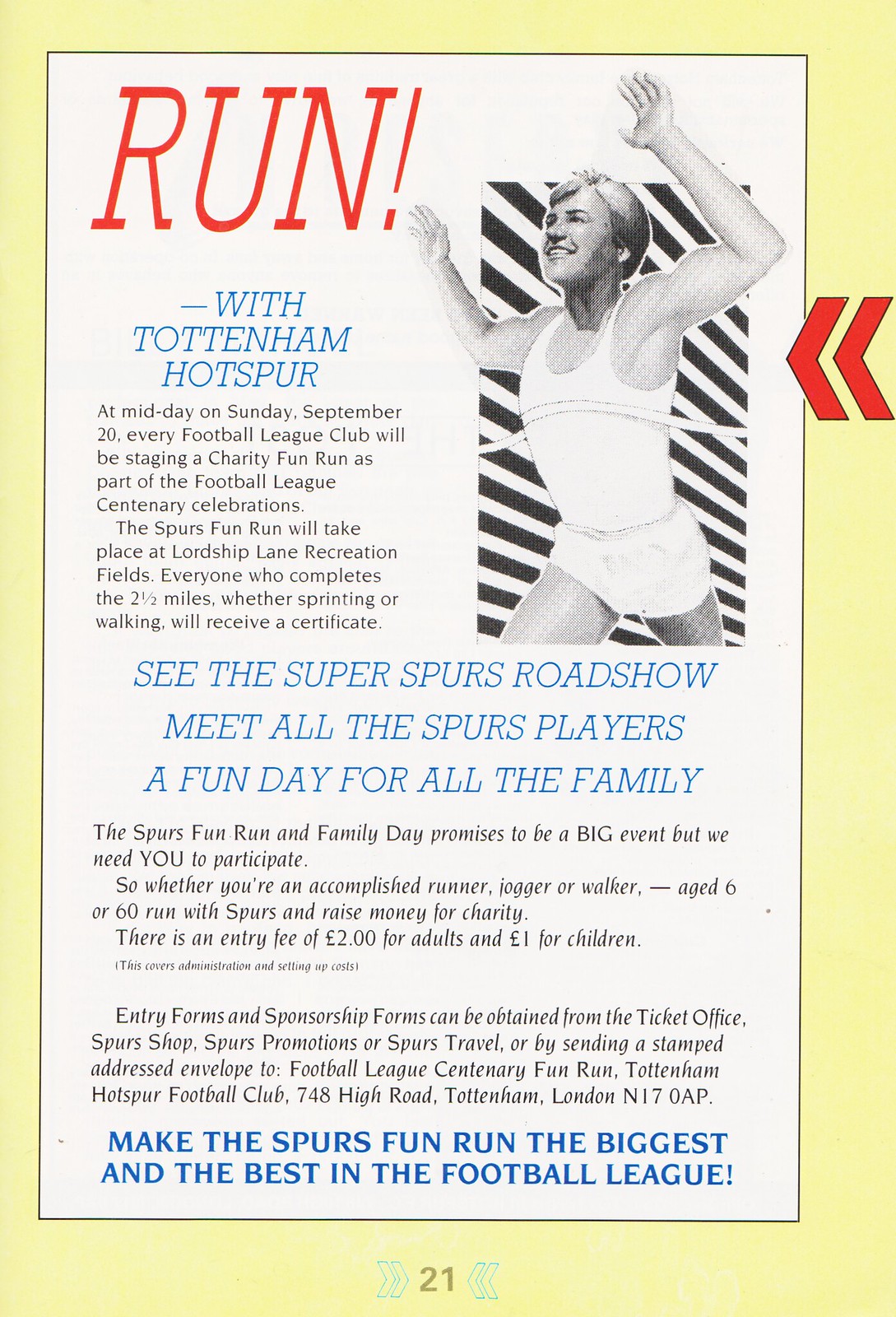A vibrant promotional banner with a yellow pane, yellow trim, and a central white rectangle outlined in black grabs the reader's attention. Bold red letters shout "RUN!" in the center, accompanied by a black-and-white drawing of a runner breaking through a finish line, clad in a white tank top and shorts. The dynamic image is enhanced by two red arrows pointing towards the runner, who is surrounded by diagonal black and white lines. Below "RUN!," white and blue text states, "Run with Tottenham Hotspur."

A detailed article reveals that at midday on Sunday, September 20th, all college leagues will stage a charity run to celebrate the Football League's centenary. Participating in the Spurs Fun Run at Lordship Lane Recreation Fields promises a certificate for everyone completing the 2.5 miles, whether they sprint, jog, or walk. Blue capital letters encourage attendees to "SEE THE SUPER SPURS ROADSHOW," meet all the Spurs players, and enjoy a fun day for the family. Complementing this, black text emphasizes the grand scale of the event, urging all to participate regardless of age or fitness level.

The event fee is $2 for adults and $1 for children, covering administrative and setup costs. Entry and sponsor forms can be obtained from the Spurs' ticket office, shop, promotions, and travel offices or by sending a stamped addressed envelope to Football League Centenary Fun Run at Tottenham Hotspur Football Club, 748 High Road, Tottenham, London, N17 0AP. The banner’s enthusiasm culminates in blue capital letters declaring, "MAKE THE SPURS FUN RUN THE BIGGEST AND BEST IN THE FOOTBALL LEAGUE," and is rounded off with the number 21 at the bottom.